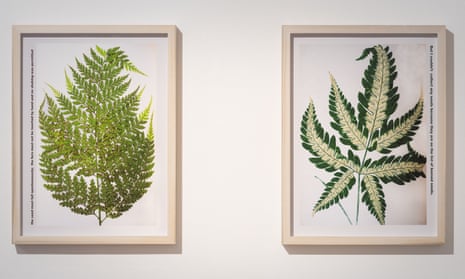This photograph features two framed images of different types of plants, each hanging on a white wall. The frames are wooden and have a vanilla or beige hue. Both plants are depicted against a white background, enhancing the vibrant colors of the leaves. 

In the frame on the left, the plant has light olive green leaves that are clustered closely together. The shape of the leaves is distinct but difficult to describe precisely. The image includes small, barely discernible writing that runs vertically from the bottom to the top of the left corner of the frame.

The frame on the right showcases a different plant species. Its leaves have a striking color gradient, with dark green edges that transition to a light yellow center, forming a star-like shape. The leaves are more spread out compared to the left image. Similar to the left frame, there is fine vertical writing on the right edge, which is hard to read due to its small size.